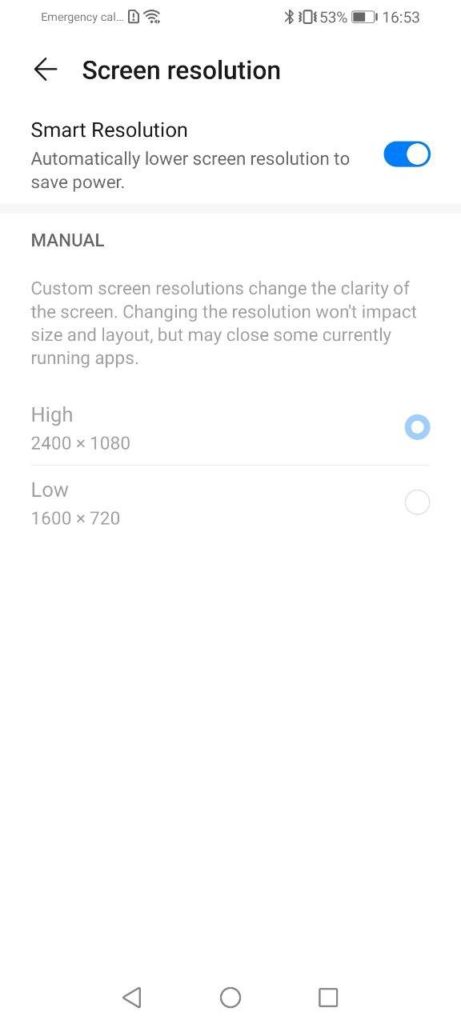The image depicts a smartphone screen displaying the settings menu with specific focus on screen resolution options. At the very top left corner, there's an "Emergency Call" icon alongside the phone's signal bars. On the right side, the battery icon indicates a 53% charge and the time is shown as 16:53.

Below the status bar, in bold black text accompanied by a backward arrow icon, the heading "Screen Resolution" is visible. Directly beneath, "Smart Resolution" is listed, with a description in gray text stating, "Automatically lower screen resolution to save power." An adjacent blue and white toggle switch indicates this feature can be turned on or off.

A small gray bar separates this section from the "Manual" option, marked in a gray-black font. This section explains, "Custom screen resolution change. Changing the resolution won't impact size and layout but may close some currently running apps."

Below this explanation, two specific resolution options are listed. The first option, "High 2400 x 1080," is selected and highlighted in blue. Following this, a gray bar separates the second option, "Low 1600 x 1720," which remains unselected, indicated by an unchecked circle to its right.